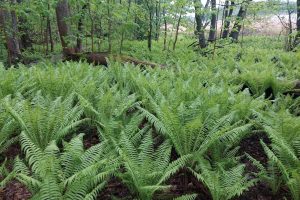The image showcases a verdant field filled with green ferns, sprawling uniformly across the ground almost to the top of the frame. These ferns, interleaved closely together, appear well-tended and healthy, with vibrant leaves reaching about a foot in height. Interspersed among the ferns are several trees; some standing tall with slender trunks crowned with green leaves, while on the left side, a fallen tree trunk lies on the ground. The background reveals a scenic gradient: a distant tree line bathed in a mix of white-blue sky and tan hues, potentially signifying additional vegetation or bushes, punctuated by glimpses of rolling hills on the right. Toward the top right corner, the sky peeks through, adding a celestial touch to this natural tableau. The ground beneath the ferns seems to be covered in bark or compost, giving the scene a well-maintained, almost cultivated appearance.